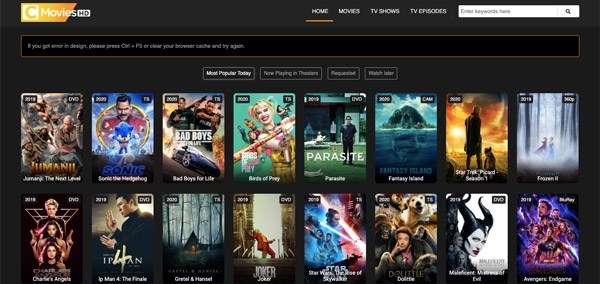A detailed caption for the described image could be:

"Screenshot of a movie streaming website's interface with a dark gray or black background. At the top-left corner, the word 'Movies' is prominently displayed, accompanied by a small white 'HD' box. Below these, there is a search bar for user queries. The top row of movie thumbnails includes titles from left to right: 'Jumanji: The Next Level,' 'Sonic,' 'Bad Boys for Life,' 'Birds of Prey,' 'Parasite,' 'Fantasy Island,' 'Star Trek' (specific iteration not visible), 'Frozen 2,' 'Charlie's Angels,' 'IP Man 4,' 'Gretel and Hansel,' 'Joker,' a 'Star Wars' title, 'Dolittle,' 'Maleficent,' and 'Avengers: Endgame.'"